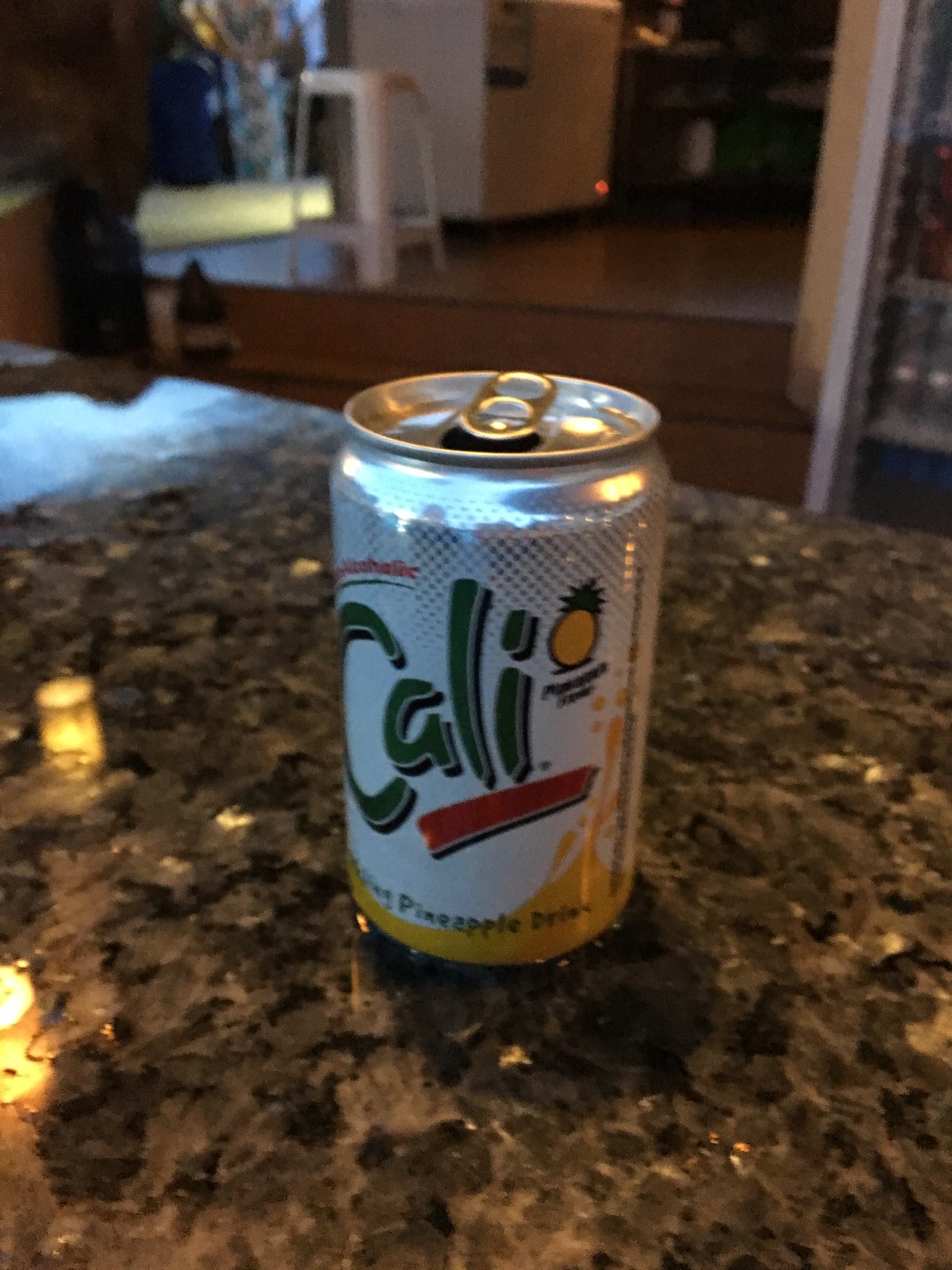The photograph showcases a close-up of an aluminum can prominently displayed on a dark, granite countertop with subtle muddy brown and greenish hues. The can itself is mostly white, adorned with vivid green lettering that spells "Kali," underlined by a sleek red line. Above the brand name, in smaller red letters, the can reads "non-alcoholic." A stylized image of a pineapple graces the lower section of the can, which also features a blend of yellow at the base and the text "sparkling pineapple drink."

In the background, slightly blurred, the scene appears to be taken inside a house. There's visible wooden flooring and a pair of steps leading up, possibly indicating a sunken kitchen design. Additional background elements include a white stool and what might be a drink cooler to the left of the steps. A jar or bottle is perched on the steps, and a white refrigerator is faintly visible. The top of the can catches some light, making it challenging to discern if it is silver or gold. The overall focus remains sharply on the can, amidst the softly illuminated backdrop.